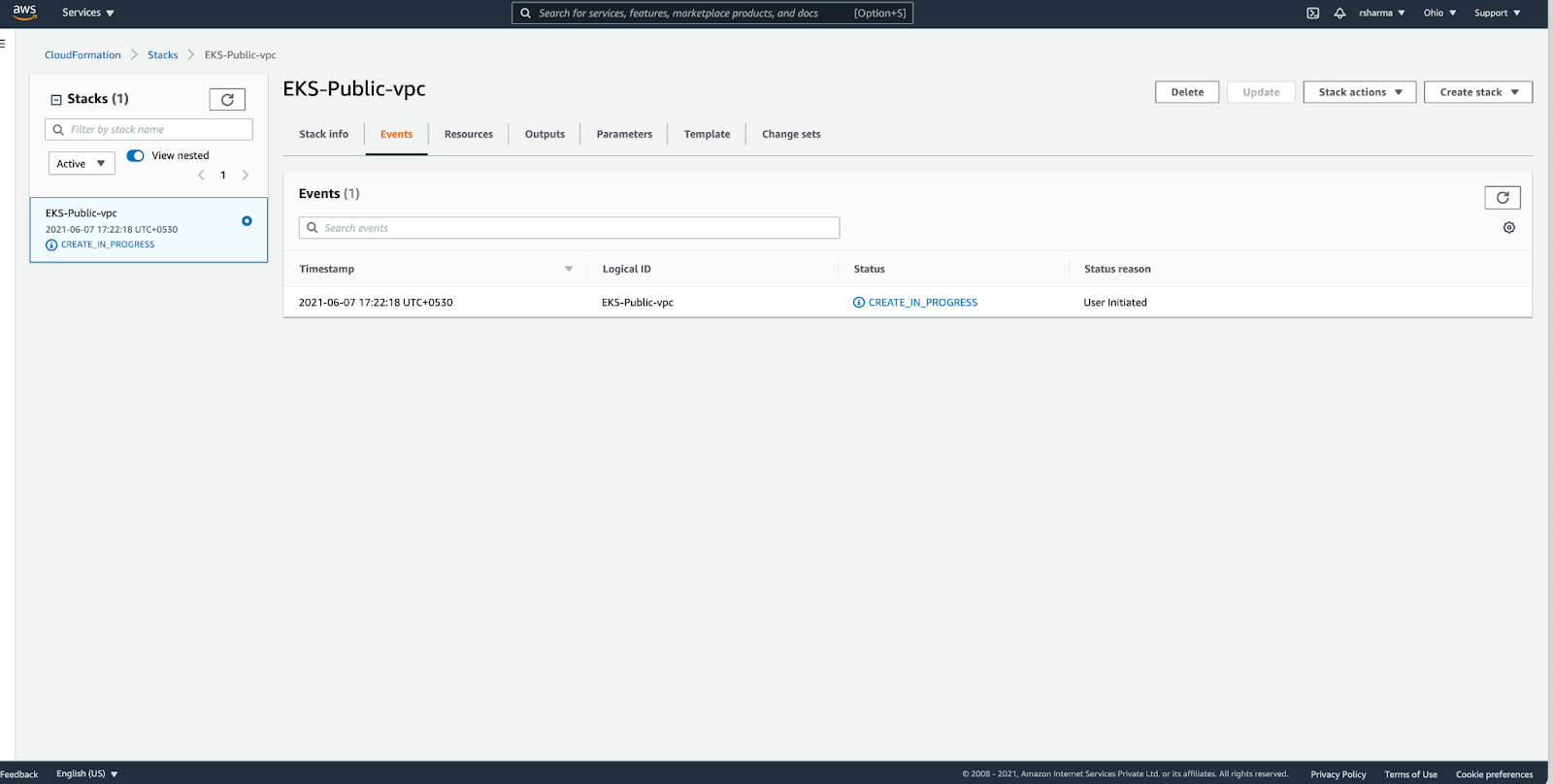Screenshot of an AWS (Amazon Web Services) Administrator Dashboard focusing on CloudFormation Stacks in the Ohio Service Region. The interface displays a single CloudFormation stack labeled “EKS-public-vpc,” indicative of a virtual private cloud setup. On the left-hand side, the sidebar showcases settings and a navigation panel emphasizing "Stacks," with the EKS-public-vpc stack highlighted. 

On the primary section of the dashboard, under the header “EKS-public-vpc,” a detailed table is presented, listing various events associated with the stack. This table comprises columns for ‘Timestamp,’ ‘Logical ID,’ ‘Status,’ and ‘Status Reason.’ There is one recorded event:
- Timestamp: 2021-06-07 17:22:18 UTC+05:30
- Logical ID: EKS-public-vpc
- Status: CREATE_IN_PROGRESS
- Status Reason: User Initiated

This snapshot succinctly captures the ongoing process and status of the stack creation within AWS CloudFormation for efficient virtual private cloud management.